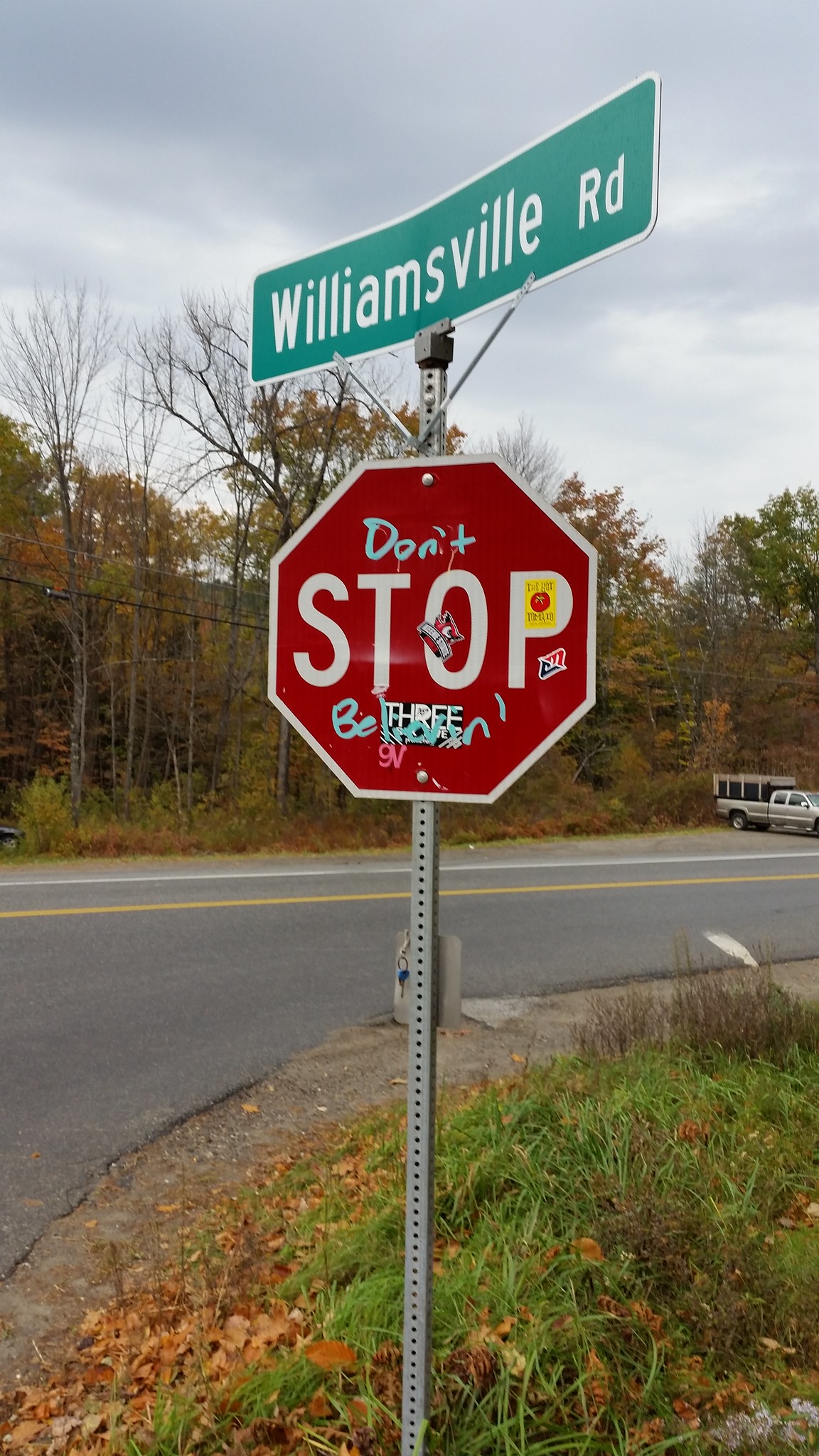The color photograph, taken outdoors in portrait mode, captures a detailed street scene focused on a stop sign with graffiti. The red, hexagonal stop sign, bordered in white and displaying the word "STOP" in white block letters, has been defaced. In light teal mint blue paint, the word "DON'T" is inscribed above "STOP." Below "STOP," the words "BE" and an illegible phrase are visible due to being partially covered by additional graffiti and a black sticker with a white "3." An additional small "PM" sticker is affixed to the right side of the sign, with a yellow sticker partially obscuring the "P." The stop sign is mounted on a pole beneath a street sign for "Williamsville Road," written as "RD." The background features a curved gray asphalt road and some trees, suggesting the photo was taken at a street corner.